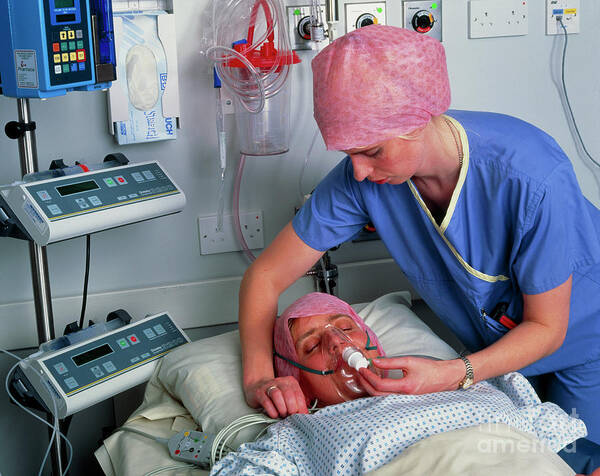In a brightly lit hospital room, a nurse dressed in blue scrubs and a pink hair cap is attentively adjusting the oxygen mask on an unconscious female patient, who is lying in a hospital bed. The patient, wearing a hospital gown and a matching pink head covering, appears to be asleep with her eyes closed and her face flushed. The nurse, who has a wedding ring and a watch on, is carefully securing the oxygen mask, ensuring the patient’s comfort and safety. To the left, a medical machine with wires and tubes monitors the patient's vitals. The wall behind them is equipped with a box of gloves, various containers, and control dials for adjusting room settings such as temperature and bed height. An outlet is also visible behind the nurse. The bed is neatly made with a pillow and sheets. The photograph, possibly intended for a medical textbook, is well-lit and includes some text at the bottom, though only partially legible, suggesting the word "Ameri-red."